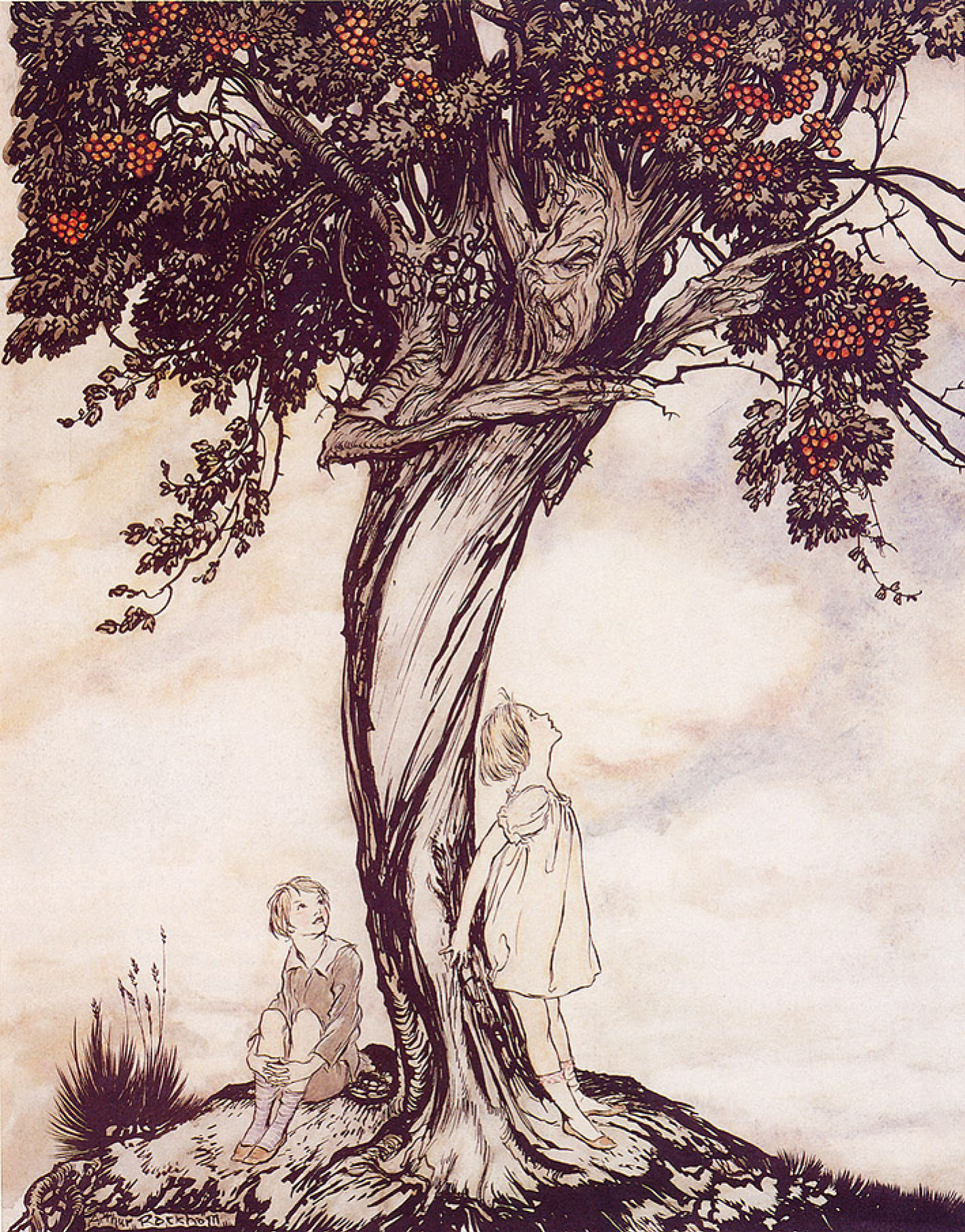The illustration, rendered in a hand-drawn pen and ink style reminiscent of early 1920s children’s books, features a fantastical scene in mostly black and white with only a few touches of color. Set on a small mound, the central figure is a large, somewhat eerie tree that intriguingly comes to life with a face and arm-like branches. The tree's face, with its long, pronounced features, looks down with a certain mysterious expression. Only the tree's clusters of bright red berries and subtle green leaves break the monochrome palette, providing vivid contrast. 

In the scene, a little girl stands with her back against the tree trunk, head tilted upwards, curiously gazing at the tree's face and placing her hand on the bark. Nearby, a little boy sits on the mound’s edge, also looking up with a sense of wonder, unafraid of the tree’s animated presence. The tree's large wooden finger points off to the right side of the image, guiding the viewer’s eye towards the upper branches adorned with red berries. The setting seems serene rather than menacing, augmented by a subdued, swirly background that merges brown and beige hues. There is a signature at the bottom left corner, too small to decipher, suggesting this could be an illustration from a children’s fantasy book.